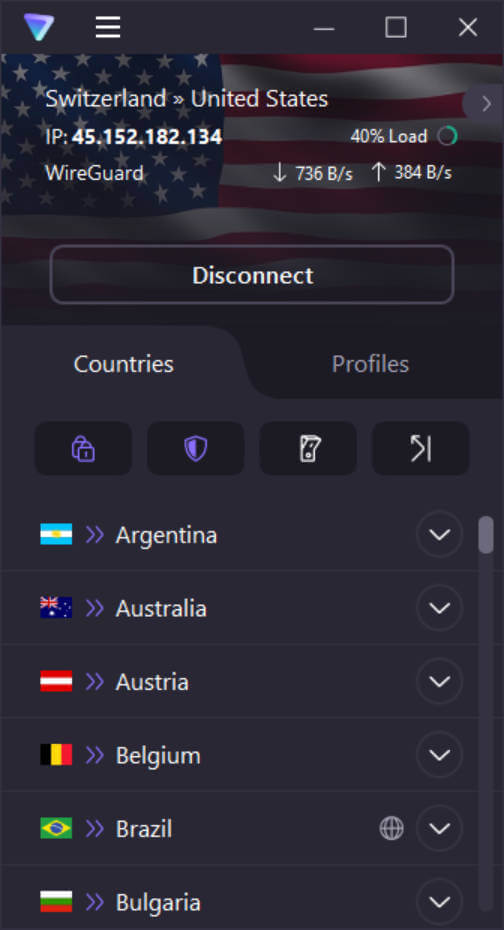This screenshot depicts a VPN interface with a dark and shadowy U.S. flag background, giving it a gray-tinted appearance. At the top, the interface shows "Switzerland" and "United States." Below those country names, it lists the IP address "45.152.182.134" with a load percentage of "40%". The VPN protocol in use is identified as "WireGuard," which has a down arrow indicating a download speed of "736 V/s" and an up arrow showing an upload speed of "384 V/s." A large rectangular "Disconnect" button is positioned beneath this information. At the bottom of the interface, there are two tabs: "Countries," which is highlighted, and "Profiles." The highlighted "Countries" tab features four icons: a lock symbol on the left, followed by a shield, a button, and lastly, a twisted arrow with an adjacent vertical up-and-down line.